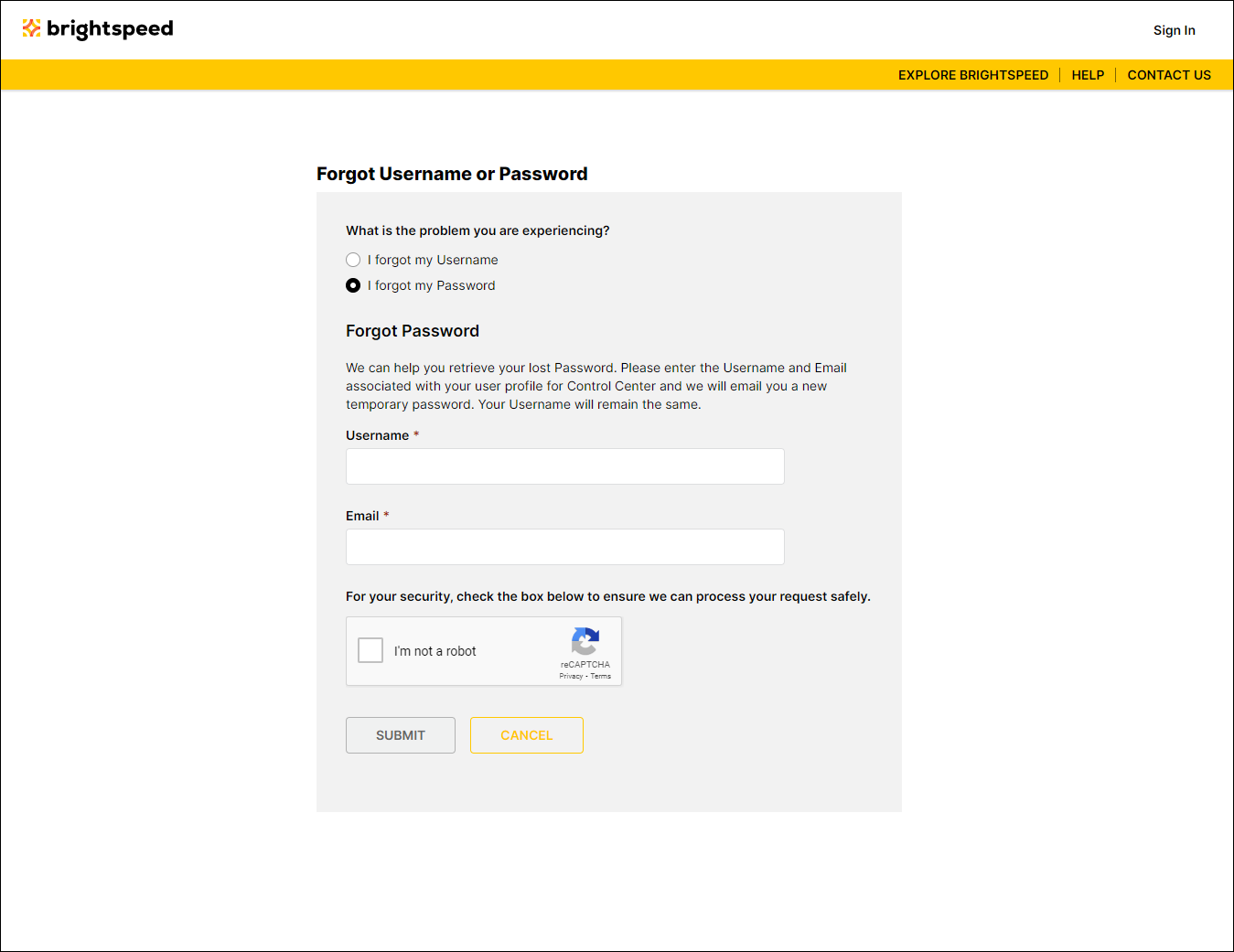The image displays a webpage from the Brightspeed website, with the logo prominently positioned at the top left corner against a yellow bar. On the top right, the site provides various navigation links, including options to "Sign In," "Explore Brightspeed," "Help," and "Contact Us."

Centrally focused, the page addresses the issue of forgotten login credentials. Text prompts users with the question, "What is the problem you are experiencing?", and the option "I forgot my password" is pre-selected. Instructions below indicate, "We can help you retrieve your lost password. Please enter your username and the email associated with your user profile for the Control Center, and we will email you a new temporary password. Your username will remain the same."

Below these instructions are fields for entering the "Username" and "Email," both currently blank and required for resetting the password. For security purposes, there's a checkbox labeled, "I'm not a robot," accompanied by a reCAPTCHA privacy terms link. At the bottom, the user is given two action buttons: "Submit" in gray and "Cancel" in yellow.

The color palette of the webpage includes accents of yellow, black, blue, and gray set against a clean white background.